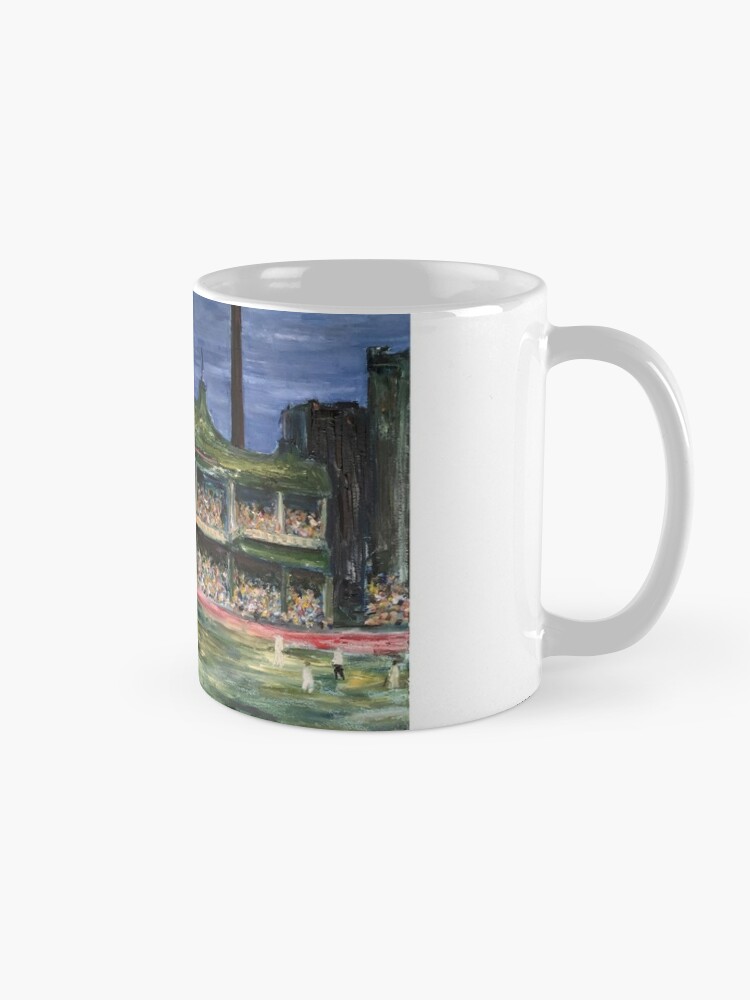This image features a white ceramic coffee mug set against a pristine white background, as if carefully staged in a studio. The mug, shown in a side profile, prominently displays a vivid and detailed art print on its left half. The print depicts a dynamic scene of a baseball game, capturing the moment with remarkable clarity. The background of the printed image suggests a green baseball field with a player at the plate, surrounded by two-story spectator stands filled with animated fans. The sky appears in shades of blue, while red and yellow accents add depth to the vibrant outdoor scene. The mug's right half, including the handle, remains a glossy, unadorned white, contrasting elegantly with the colorful depiction beside it.